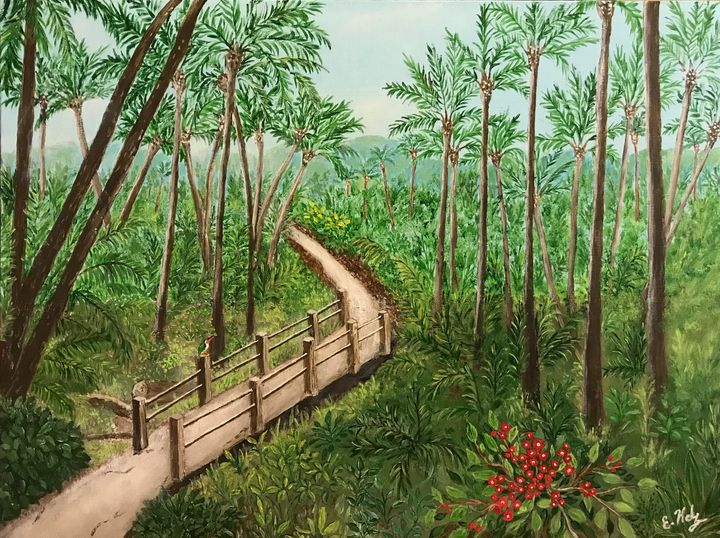The image is a detailed painting of a tropical forest clearing, featuring a long, brown dirt pathway that starts at the bottom left corner, ascends diagonally, and curves back toward the upper right. The walkway is bordered by wooden rails at certain points. The forest is dense with various tall trees, including palms, some bearing coconuts, and other lush vegetation. In the foreground, green leaves surround small, round red berries. Mountains provide a scenic backdrop to the forest setting, adding depth to the scene. The painting contains the artist's signature, "E-H-O-Y," in white cursive writing at the bottom right corner. The lush greenery and vivid details convey a sense of serenity, reminiscent of a tropical paradise like Hawaii.